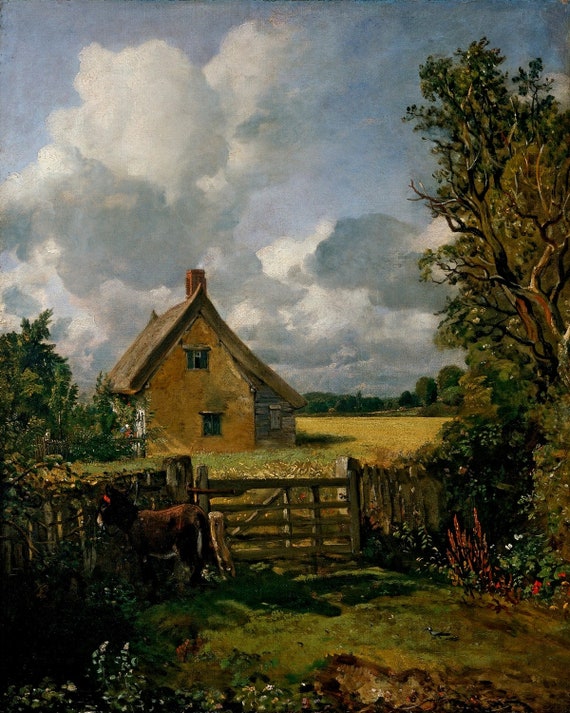The image is an old oil painting depicting a quaint 19th-century farmhouse. The two-story farmhouse features a brown exterior with one end showcasing red brick. The roof, which is gray and peaked, slopes more sharply on the right side, sheltering a wooden shed or root cellar beneath. The front of the house displays a couple of windows and is framed by a vibrant green grass, interspersed with hints of brown, indicating its health.

In the foreground, a brown wooden fence encircles the property, adorned with vines and backed by a grassy path. A small brown mule, identifiable by its white snout and a red tag in its ear, stands outside this fence, seemingly nibbling on flowers. To the left of the house, lush vegetation and trees are present, while more trees with green leaves and brown trunks populate the right side of the image.

The landscape stretches into a large field with a yellow hue, flanked by a line of distant trees. Overhead, the sky is a blend of blue and white clouds, giving a sense of a cloudy day. The painting is rich in detail, capturing the essence of a serene, historical rural scene.